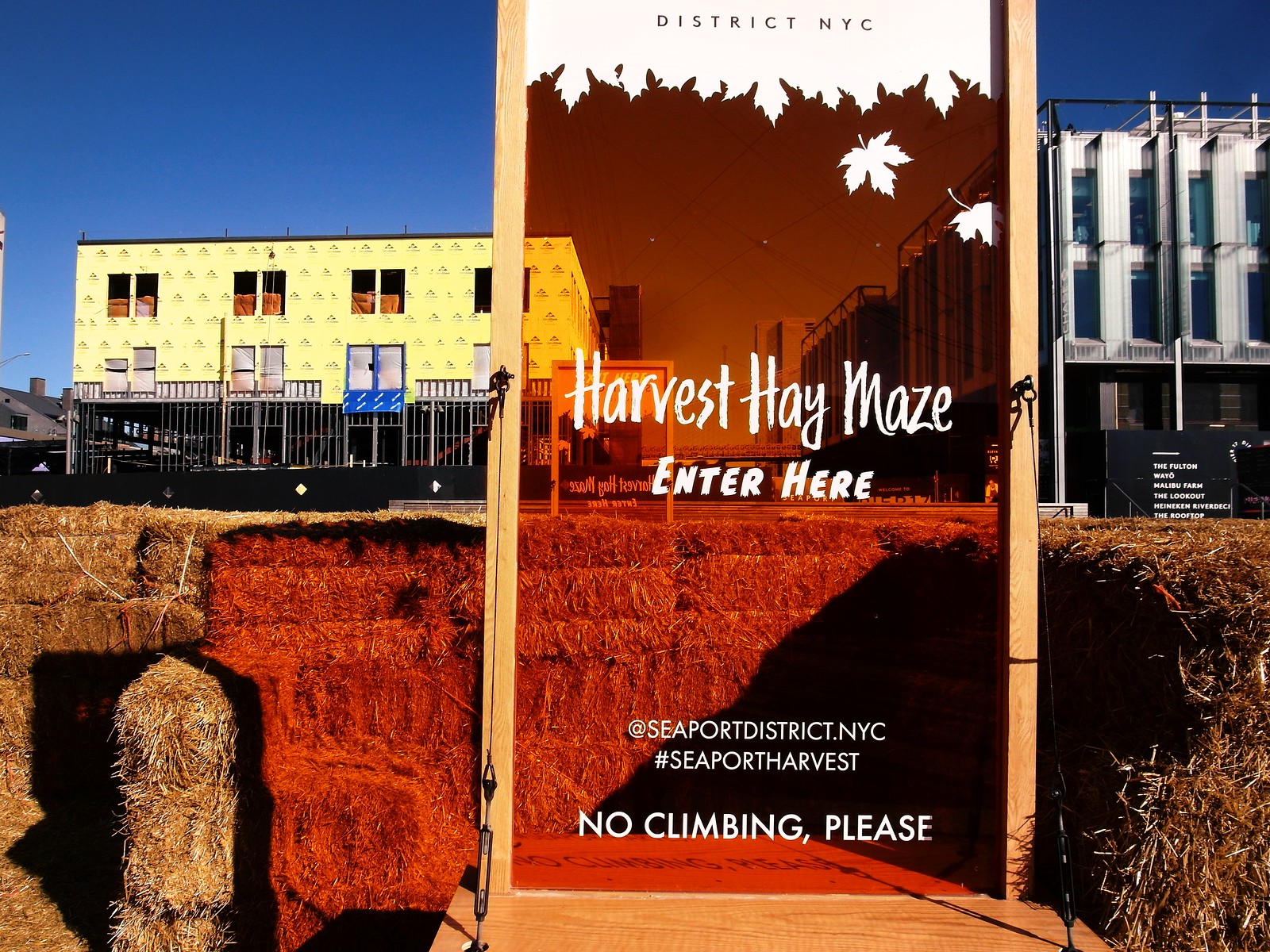The image appears to be an advertisement for a Harvest Hay Maze at the Seaport District in NYC. The sign is set within a transparent or semi-transparent glass or acrylic frame, featuring an orange background with white lettering that reads "Harvest Hay Maze Enter Here" and "Seaport District NYC #SeaportHarvest." Additionally, there's a reminder, "No Climbing Please." The backdrop reveals a construction site with two buildings: a modern, nearly finished building to the right and another under construction with visible insulation and ladders to the left. In front of the sign are piles of bales of hay, underscoring the maze theme. The scene is captured under a clear, blue sky with no clouds, indicating it was taken during the daytime.